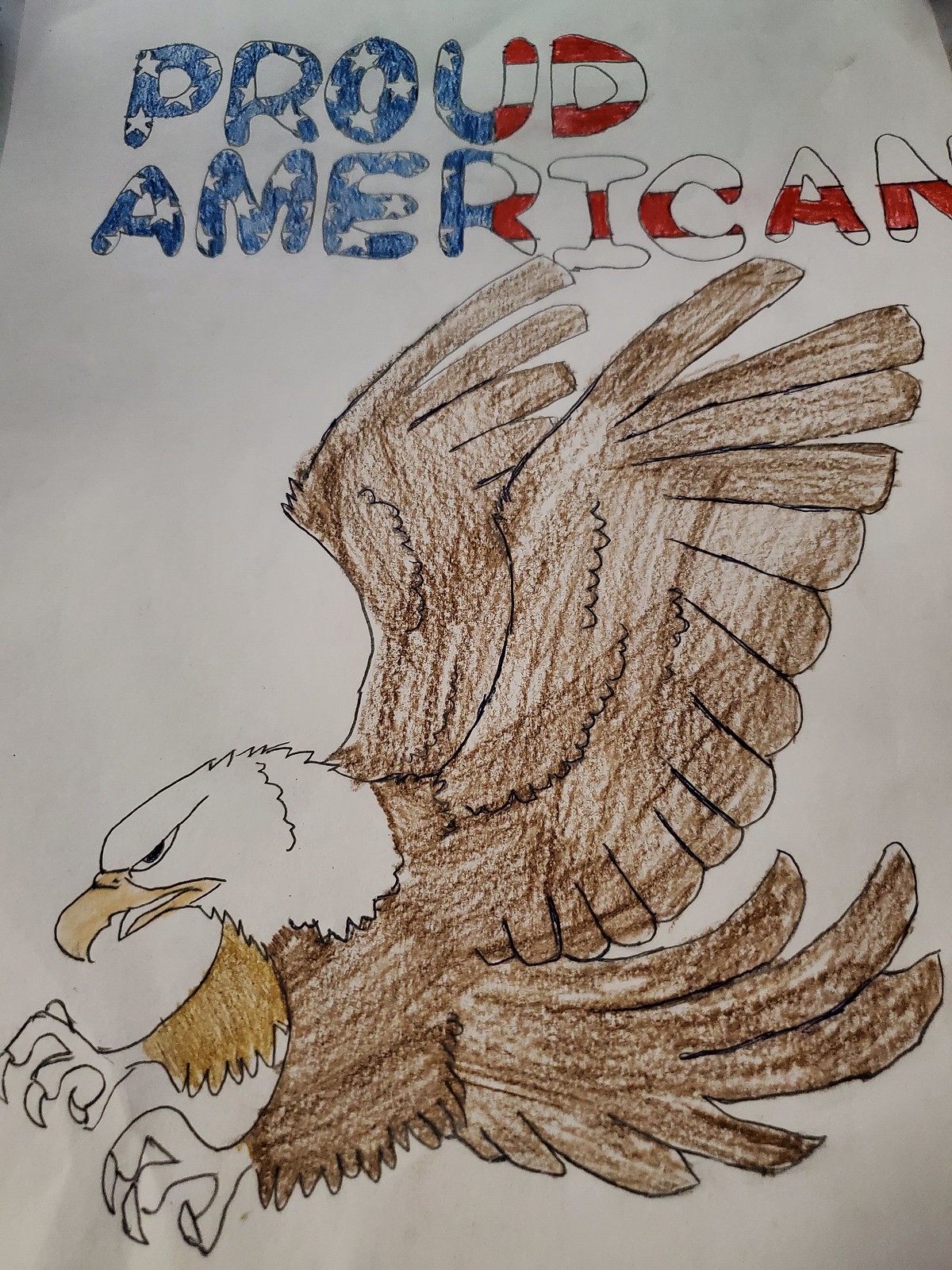This hand-drawn illustration, created in pen, prominently features the words "PROUD AMERICAN" at the top of the page. The intricate lettering combines patriotic themes, with letters P-R-O and parts of U, A-M-E, and R shaded blue and adorned with white stars, while the rest of the lettering displays striking red and white stripes. Beneath this bold text, an eagle is depicted with its wings majestically outstretched above its body, seemingly mid-flight and facing left. The eagle's outstretched talons suggest a dynamic motion of reaching or grasping. The artist has colored the eagle predominantly in varying shades of brown, except for its right leg which is a lighter brown, adding a sense of depth and detail. The eagle's beak stands out vividly, colored in a bright, contrasting yellow.